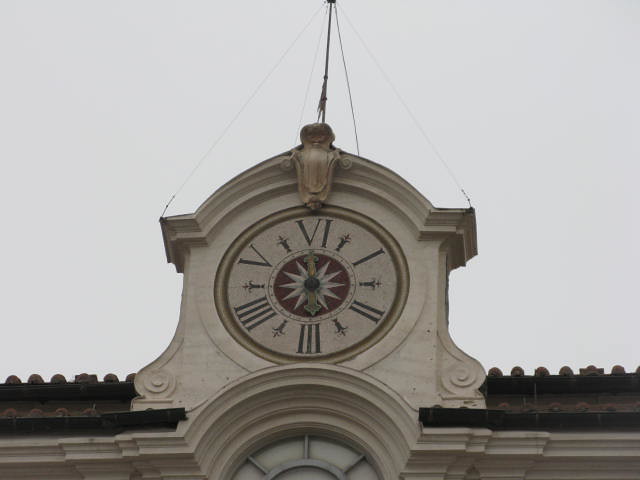This photograph captures an upward view of a clock mounted atop a building, set against a gray sky. The building's roof is adorned with black tiles, adding a stark contrast to the gloomy backdrop. Above the clock, a metal lightning rod extends upward, secured by lines that stabilize it against the clock's structure. The clock itself is encased in a frame characterized by straight lines on each side and a domed, rounded top. 

The clock face is circular, adorned with Roman numerals. However, the numerals appear to be inaccurately positioned, with "VI" at the top and "III" at the bottom, contrary to the conventional arrangement. A distinctive feature of the clock is the red circular detail at its center, emblazoned with a white star. This central motif adds an unexpected splash of color and uniqueness to the otherwise traditional timepiece.